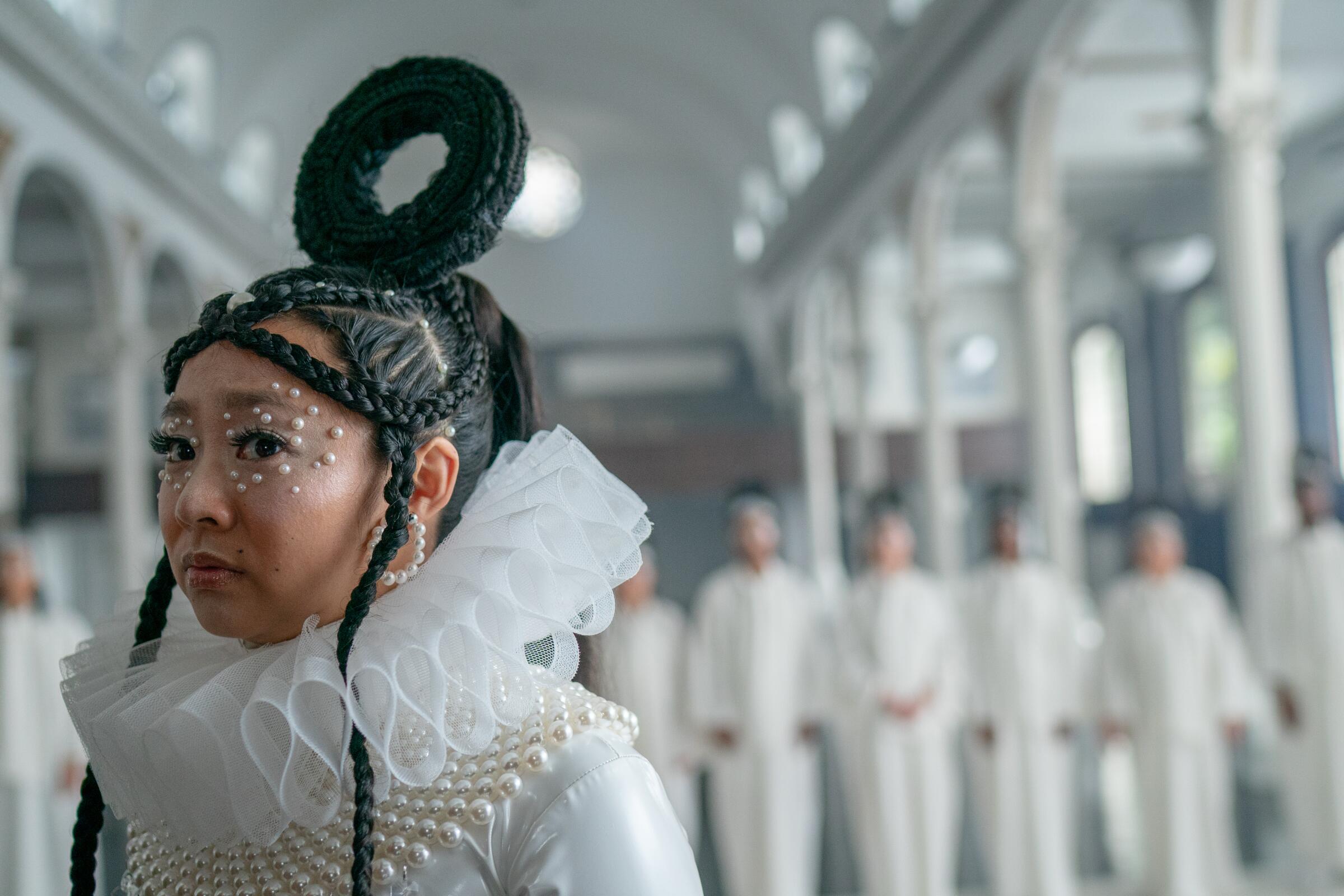This highly detailed close-up photograph captures a young woman of Asian descent, adorned in an elaborate and ornate costume exuding a distinct regal aura. Her hair is styled into numerous braids, including a prominent circular braid on top of her head, reminiscent of a donut shape. Her black hair frames her almond-shaped eyes, which are intricately decorated with encrusted pearl-like jewelry and rhinestones, adding to her ornamental look. She wears an opulent chest piece composed of strings of pearls that wrap around her shoulders and chest. A striking white frilled collar reminiscent of historical royalty adorns her neck, resembling the Elizabethan ruffs associated with the era of Henry VIII. The background features a blurred assembly of individuals clad in white, standing against what appears to be the interior of a grand, white palace. Despite the rich embellishments and the grandeur of her attire, the woman wears a worried expression, adding a layer of depth and intrigue to her character.